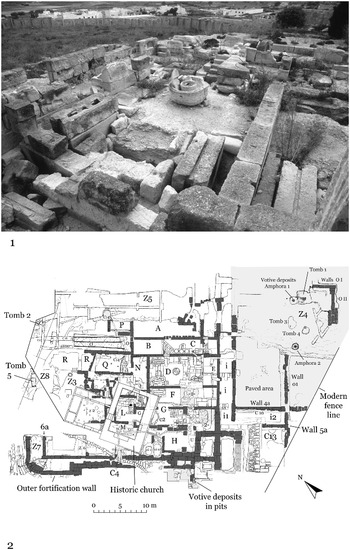The image is a composite of two black and white sections, one on top of the other. The upper half features an aerial black and white photograph of an archaeological site, showcasing a range of bricks, stones, and severely deteriorated structures that are difficult to identify. The photograph suggests a complex area filled with ancient ruins and fragmented concrete blocks. Contrasting this, the lower half presents a digitally drawn map of the same site, meticulously annotated with labels and notes. The map includes identifiers for various elements such as "Tomb 1," "Tomb 2," "Wall 1," "Wall 2," "Modern Fence Line," "Votive Deposits in Pits," "Historic Church," and various lettered sections. This detailed blueprint serves as a guide for archaeologists, highlighting the specific areas and features of the historical location depicted in the photograph above.